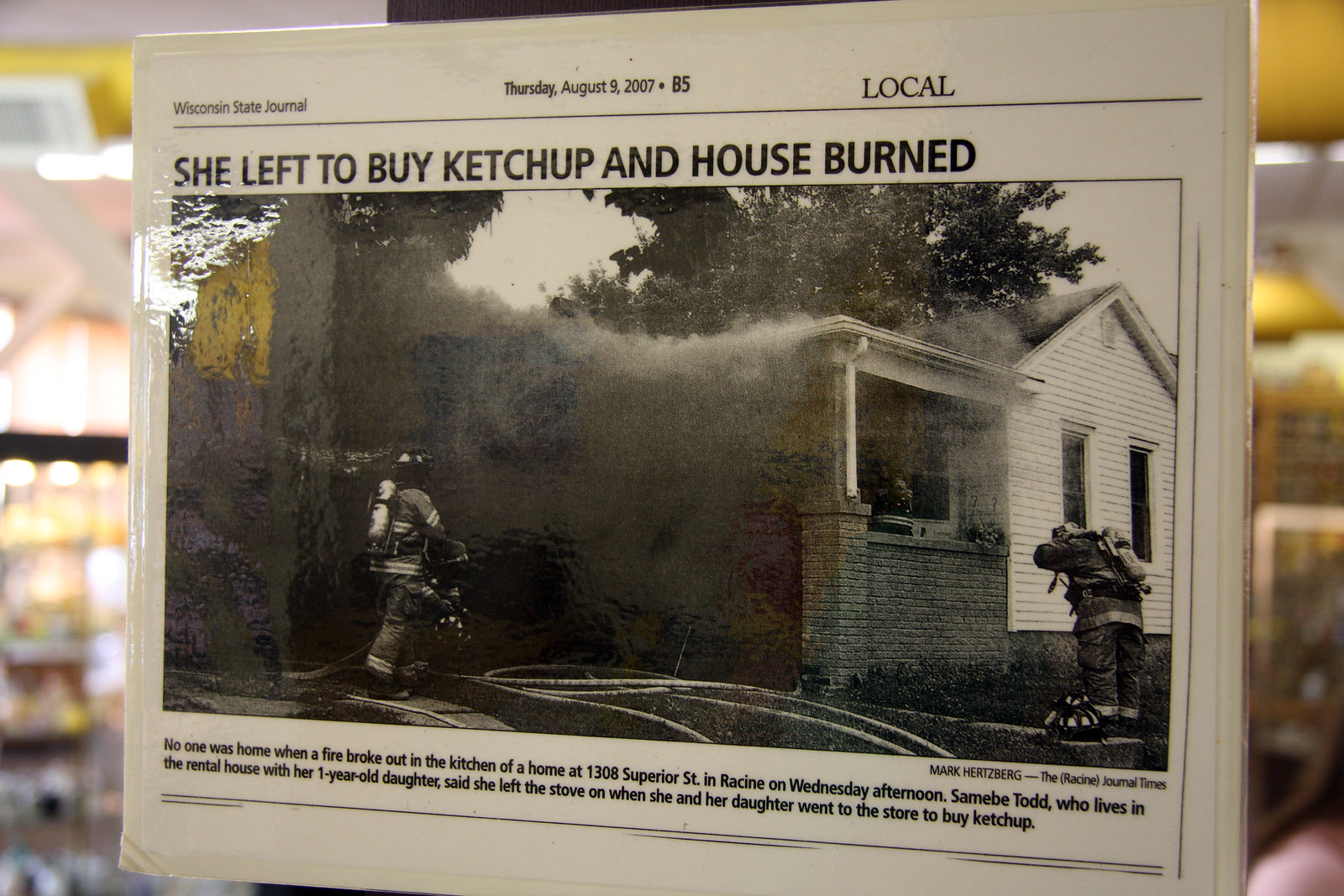This is a photograph of what appears to be a laminated sign or reproduction of a local newspaper article. The newspaper is identified as the Wisconsin State Journal, dated Thursday, August 9, 2007, on page B5. In the upper corner, it is labeled "Local." The headline reads, "She left to buy ketchup and her house burned." Below the headline is a large black-and-white photograph depicting a brick house engulfed in smoke. Smoke is visibly billowing from the front porch area, and two firefighters are seen approaching the house—one walking towards the front and another on the right-hand side. The caption beneath the photograph states that no one was home when the fire erupted in the kitchen of the house at 1308 Superior Street in Racine on Wednesday afternoon. The resident, Samba May Todd, who lives there with her one-year-old daughter, mentioned that she had left the stove on when they went to the store to buy ketchup. The setting of the image appears to be in a library, suggested by the presence of bookshelves in the background.